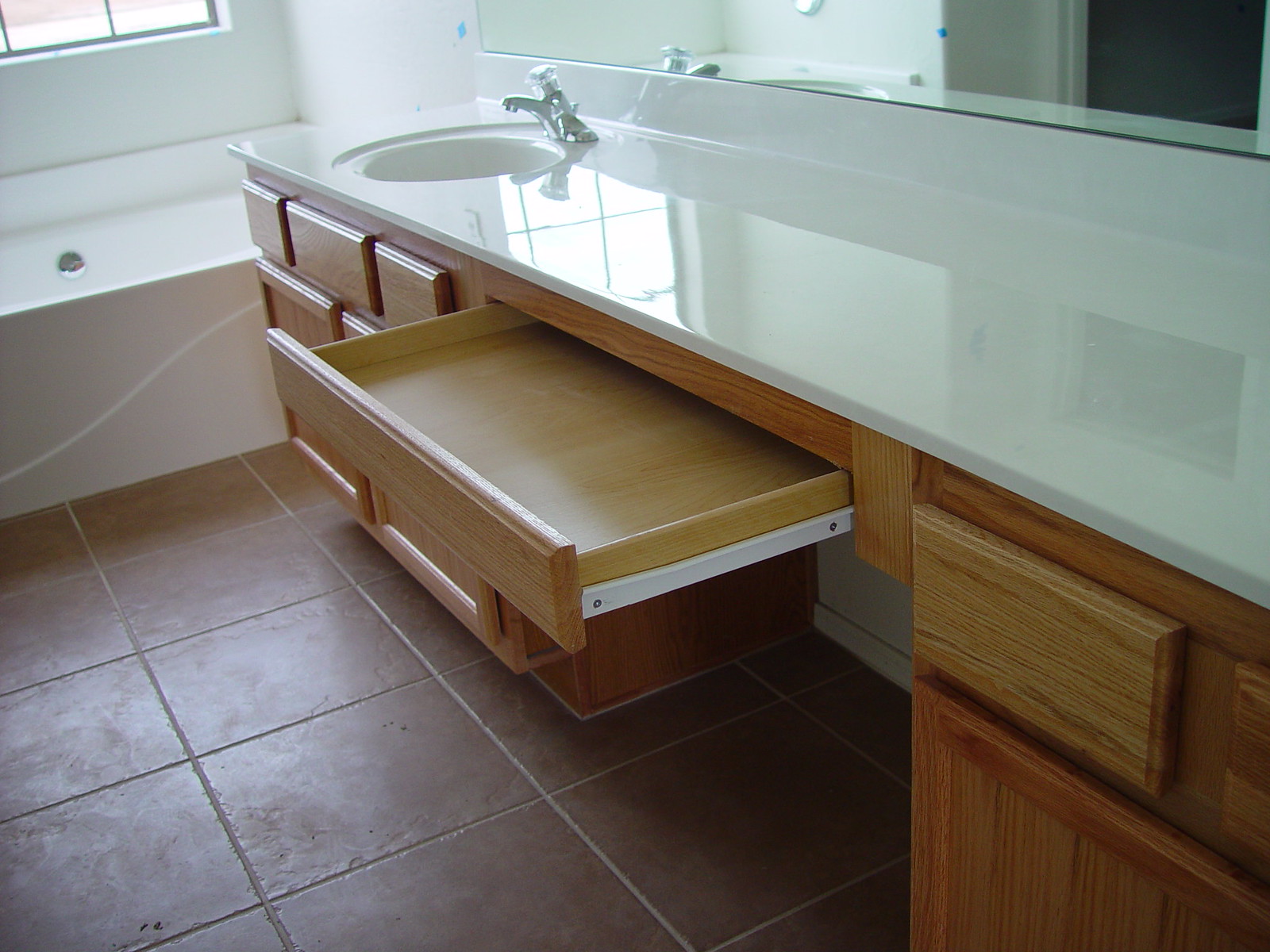The image depicts an unoccupied bathroom with a prominent view of the sink and vanity area, as well as distinct red tiled flooring. In the back right corner, there's a visible portion of the bathtub, above which is the lower section of a window with two panes. 

The focal point is the sink, which extends from the top right to the top left of the photo, set within a white tiled countertop. Below the sink, the vanity comprises three wooden drawers and two cabinets. The sink itself features a gleaming silver faucet with a single, crystal-like knob. 

Above the sink, the bottom edge of a mirror is visible. The expansive vanity extends beyond the sink, designed in three main sections. The section adjacent to the sink has an empty space underneath, reminiscent of a desk, and includes one wooden drawer that is pulled open. The final section features two more drawers and an additional wooden cabinet beneath.